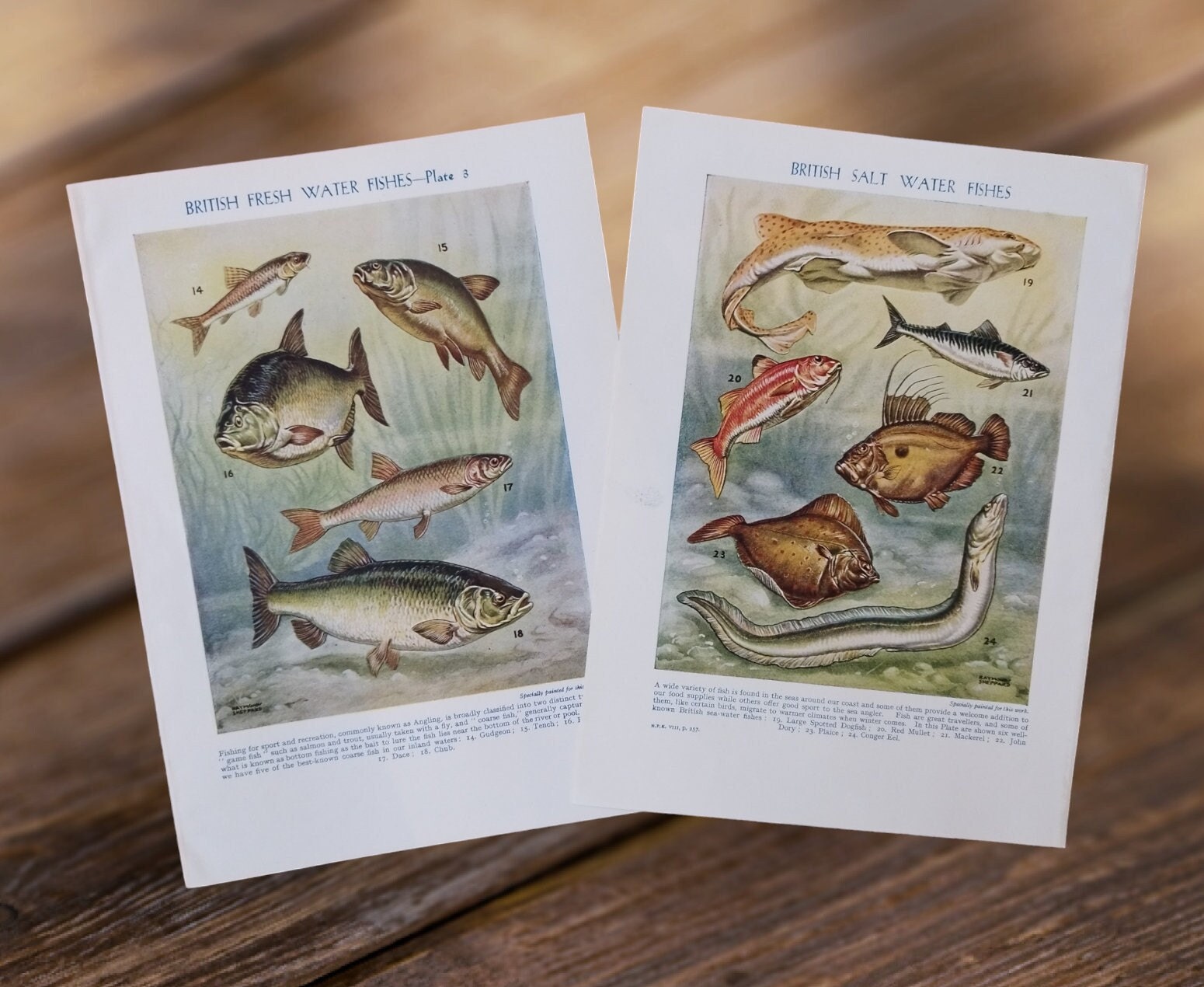This is a detailed square color photograph of two page spreads from a descriptive wildlife book, likely an encyclopedia, detailing various British fish species. The background in the image is blurred but appears to be modern wood flooring. The pages are slightly skewed, overlapping each other at the corners without obscuring any details. On the left page, titled "British Freshwater Fishes, Plate Three," five fish illustrations are displayed and numbered 14 through 18, with tiny unreadable text likely providing their common and scientific names. On the right page, titled "British Saltwater Fishes," there are illustrations of six marine creatures, including five fish and one eel, also accompanied by labels and scientific names. Both pages feature high-quality, accurate drawings that are useful for identifying these fish species, emphasizing their practical and aesthetic value.